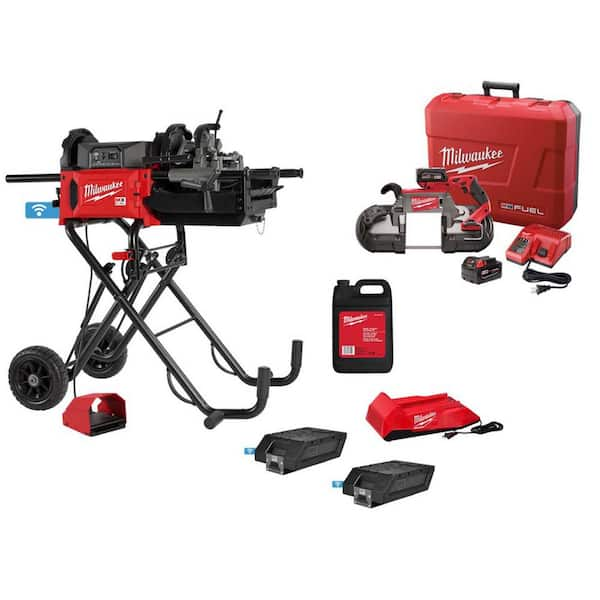This image showcases an assortment of Milwaukee brand tool sets, all prominently featuring the iconic red and black corporate colors. Positioned at the back right is a red Milwaukee tool case, adorned with the distinct white cursive Milwaukee logo and a small lightning bolt beneath it. In front of this case, there's a variety of tools and equipment, including cutting implements, a battery, a charging dock, and what appears to be a portable saw on wheels, supported by handlebars and standing upright. This saw is likely motorized, featuring a small blue block indicative of a WiFi signal, suggesting advanced functionalities. Additionally, a black gallon jug with a red label is present, possibly containing motor oil, contributing to the industrial theme. The entire setup is displayed against a pure white background, devoid of any descriptive functionality for the tools displayed.